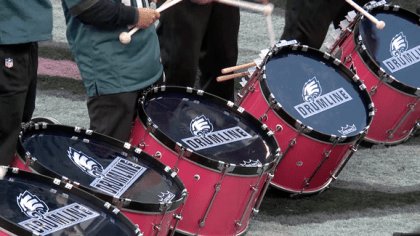This photograph captures a dynamic scene on a sports turf, predominantly green with hints of white markings forming letters or designs on the field. At the forefront are five large marching band drums, striking in their vibrant red sides and contrasting black tops and rims. Each drum is adorned with a detailed eagle head logo above a bold white stripe, inside which the word "Drumline" is spelled out in black letters. The drums are supported by silver metal components, and the players' hands are in motion, creating a slight blur. The drum carriers, visible from the torso down, are outfitted in coordinated black pants and green jackets, gripping tan or white mallets used to play the drums. The scene suggests an energetic performance by the marching band's drumline, set against the backdrop of a meticulously maintained field.